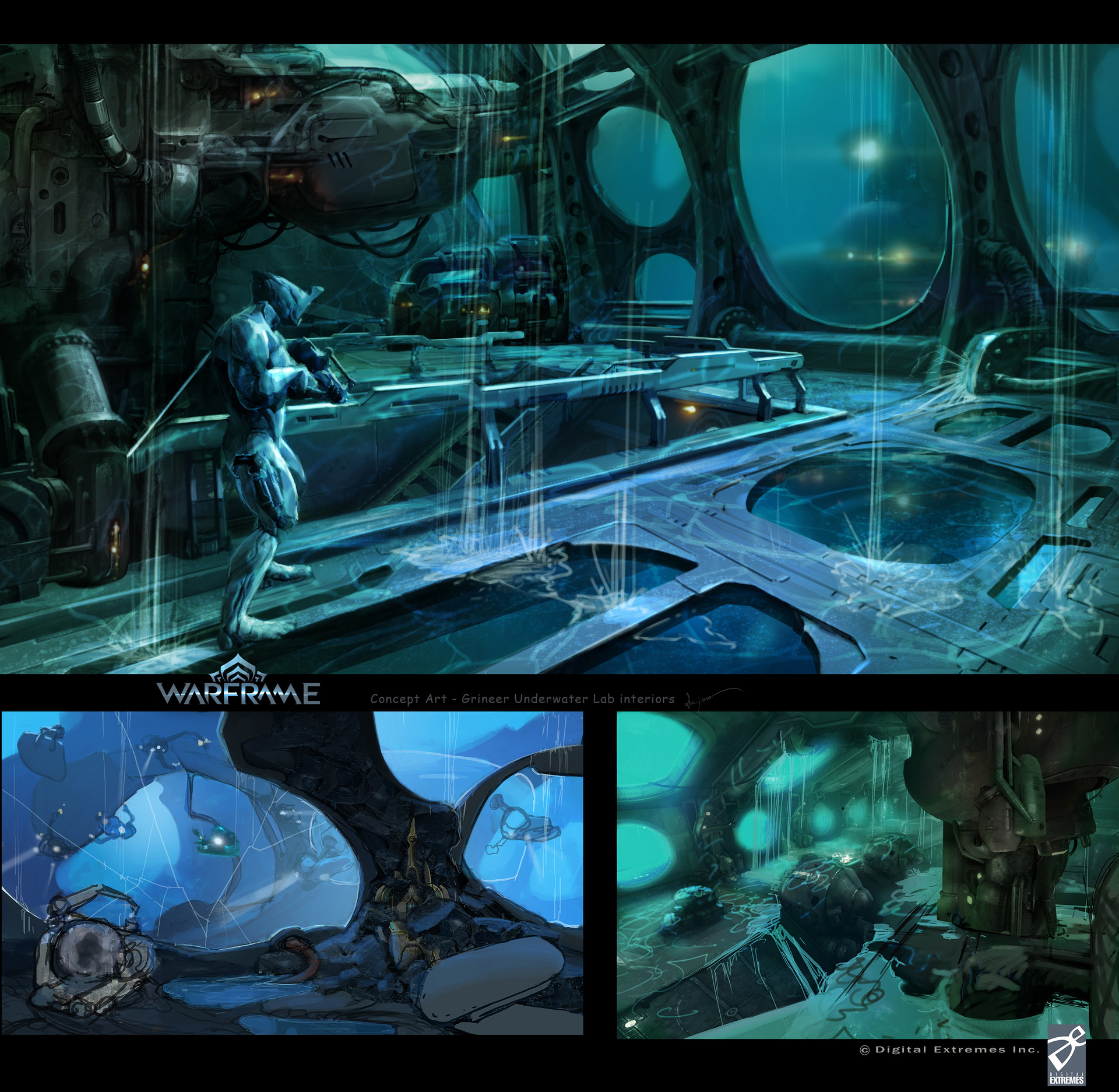The image is a detailed piece of digital animation concept art for the video game Warframe, presented as a triptych with three sections. The top section is a large, elaborately drawn scene set in a futuristic underwater environment. Dominated by tones of silvery blue to cyan, it features a possibly half-robotic character holding a gun, with water pouring in from above, suggesting a compromised submarine-like structure. This sci-fi setting displays cracked windows through which other submerged vehicles with headlights can be seen. Below this scene, the dividing section bears the title "Warframe" in silver text on a black background. The two smaller sections at the bottom depict close-up views of the top image, each with a science fiction aesthetic featuring light blue, light green, and sea green hues. The left section shows additional detail of the underwater facility's cracked windows and external machinery or robots. The right section continues the theme with more water leakage and futuristic architectural elements. The entire composition includes a Digital Extremes Inc. copyright and logo at the bottom right.